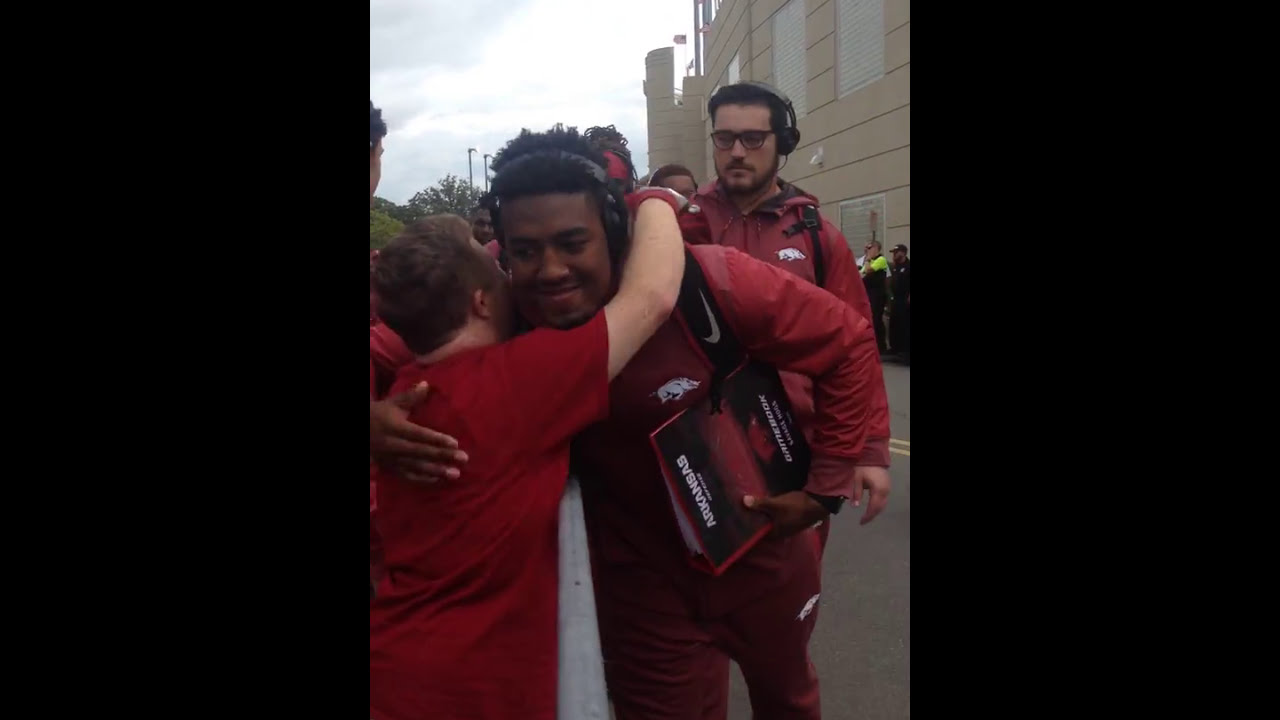In this vibrant street scene, a dark-skinned gentleman with curly black hair, dressed in a burgundy Nike jumpsuit, is stooping down to hug a young boy with light brown hair wearing a red t-shirt. The man, adorned with black headphones and a Nike backpack, cradles a red binder under his left arm, featuring a design that says "Arkansas". The little boy warmly wraps his arms around the man’s neck while they share a heartfelt moment. Behind them, another man, possibly a teammate, also in a burgundy jumpsuit with black headphones and sporting glasses with a black beard and mustache, looks on. Several more figures, partially obscured, appear in the background. The scene is set against a beige building with a blue sky and white clouds overhead, and there are trees visible to the left. The gathering, which includes a line of fans, suggests this could be a meet-and-greet possibly involving sports players.